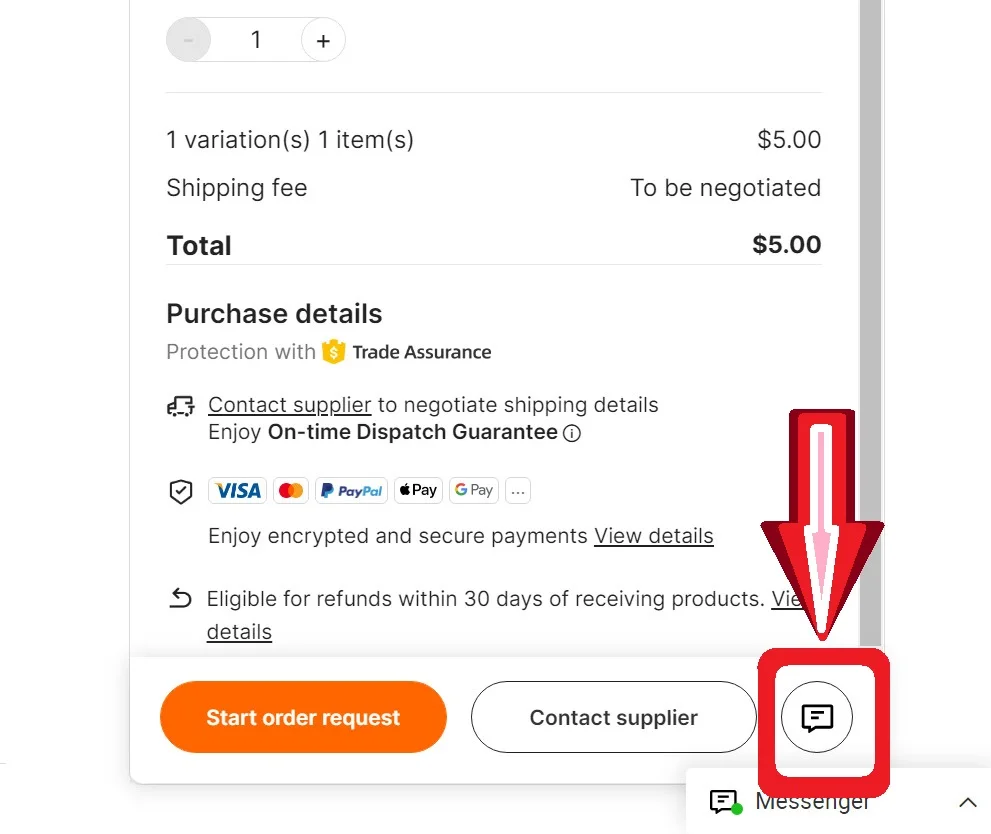The image depicts a screenshot of an online payment screen. In the top left corner, there are controls to manage the quantity of items, indicated by a "1" with a minus and plus sign, suggesting the option to add or remove items from the cart. Below this, the text "1 variation(s), 1 item(s)" is displayed, detailing the quantity and variation of the items.

On the right-hand side, the listed item has a price of $5.00. Directly beneath the quantity information, the term "Shipping fee" is noted on the left, with "To be negotiated" aligned on the right. The total amount, prominently bolded, is $5.00, aligning with the earlier price.

Separate from the main item details, "Purchase details" is written in bold, followed by "Protection with" in gray text. Adjacent to this, a gold crown emoji with a white dollar sign in its center is displayed, signifying "Trade Insurance," which is also emphasized in bold text.

Additionally, beneath the insurance information is an underlined prompt "Contact Supplier," urging users to negotiate shipping details and benefit from on-time dispatch guarantees, marked with an informational icon.

A large, multi-layered red arrow points downward, drawing attention to a message icon framed within a red box, likely indicating a help or messaging button. This arrow features dark red on the outside, a brighter red interior, followed by white and pink layers.

At the bottom of the screen, in the same row, options include "Start Order Request" on the left in orange and "Contact Supplier" presented in an oval-shaped white button with black text.